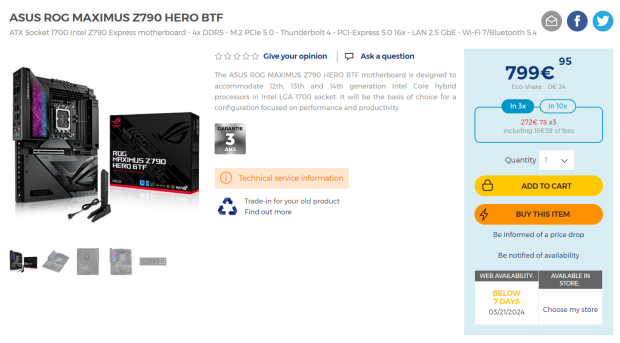**Descriptive Caption:**

At the top of the image, the background features a white and black gradient design. On the left-hand side, bold text reads "ACES, VOG, Maximus, Z790, Hero, BTF." Directly below, it lists essential specifications: "ATX, Saga 1700, Intel Z790, Express Motherboard - 4X DDR5-M, PCIe 050, Thunderbolt 4, PCI Express 5.0 16X, 2.5 GBE, WiFi 7, Bluetooth." The image shows that the product is unrated, with five empty stars outlined in black and blue. 

Highlighted in blue text is a prompt: "Ask a Question." Below this, in a detailed description, it specifies that "The ACES, VOG, Maximus, Z790, Hero, BTF Motherboard is designed to accommodate 12th, 13th, and 14th generation Intel Core Hybrid Processors with Intel LGA 1700 Socket. It is optimized for configurations focused on performance and productivity."

In the image's lower segment, there's a silver-gray square with an indistinct black word that blurs when zoomed in, followed by the number 3. Below this, there's additional text, potentially reading "ANS" or "AHS," and an orange section stating "Technical Service Information."